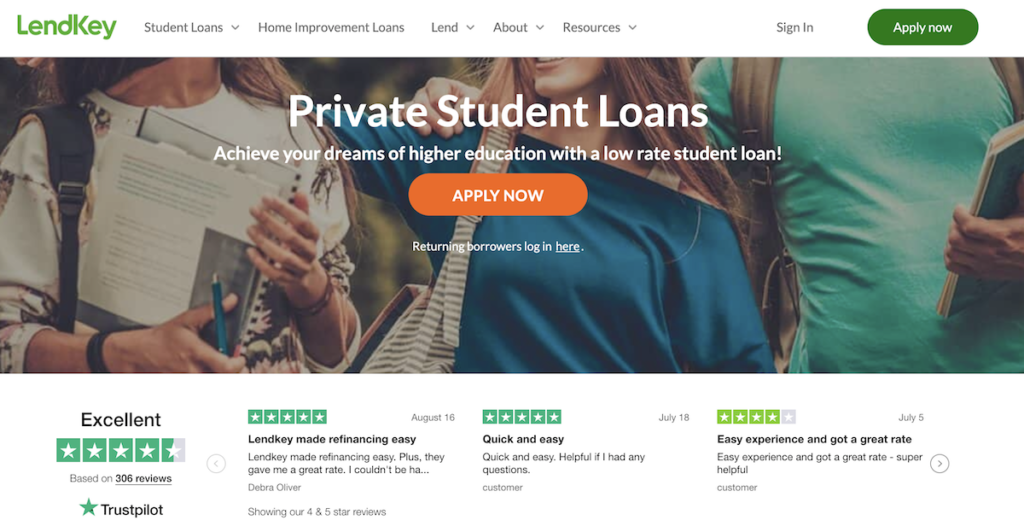A meticulously cropped screenshot of a website's home page, devoid of any web browser interface, showcases the main features of LendKey's online presence. In the top left corner, the company's logo, "LENDKEY," is prominently displayed in green text. The top navigation bar offers dropdown menus for "Student Loans," "Home Improvement Loans," "Lend," "About," and "Resources." In the top right corner, users are presented with a "Sign In" option alongside a green "Apply Now" button.

Centrally featured is a photograph of three individuals who appear to be students, holding books and carrying bags over their shoulders. Superimposed on this image is text promoting private student loans, accompanied by an orange "Apply Now" button.

Beneath the main image, the website displays four distinct reviews, each featuring a star rating, written descriptions, and the date the review was posted.